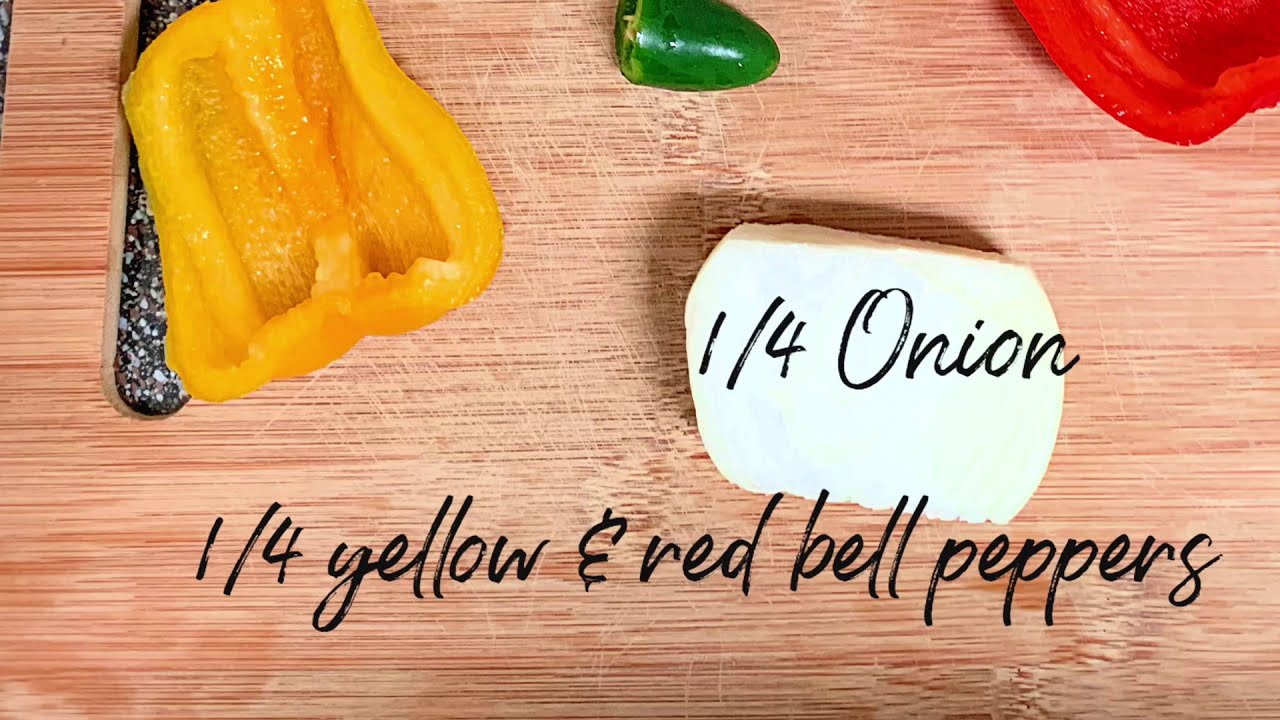This detailed image depicts a well-worn, light brown wooden cutting board covered in variously colored vegetables. Prominent on the cutting board is text written in black cursive handwriting, which serves as a recipe guide. The text "1/4 onion" is positioned centrally, while "1/4 yellow and red bell peppers" appears towards the bottom. Visible on the cutting board are a partly sliced white onion, a halved yellow bell pepper on the left, and a sliced red bell pepper peeking out from the top right corner. Additionally, a small nub of a green jalapeno is noticeable towards the top center. The cutting board showcases numerous striations and cut marks, particularly in the middle, highlighting its frequent use. A black-handled utensil extends into the frame from the upper left corner, suggesting active meal preparation. Overall, this image captures the ingredients and process steps for a colorful vegetable recipe laid out on a seasoned cutting board.